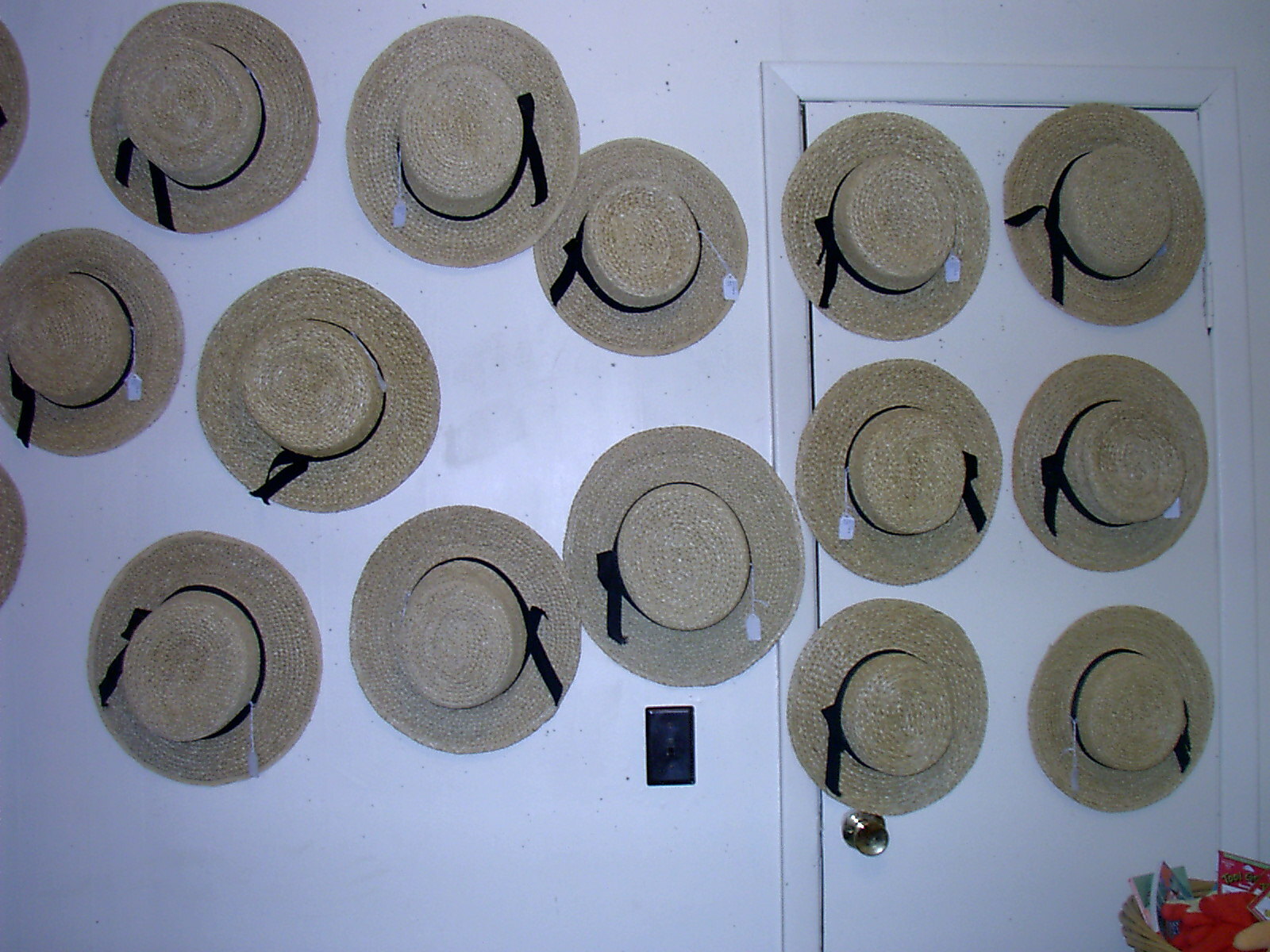This color, landscape-format photograph features a white room where numerous straw hats are creatively displayed. The hats, resembling Panama hats, are scattered across a white wall and a white, right-sided door with a brass doorknob and a black light switch beside it. Each hat is adorned with a black ribbon band tied in a bow around its base and bears a distinct white price tag, suggesting they are for sale. On the wall, the arrangement appears somewhat disorderly, adding an interesting touch of randomness, while six hats are neatly positioned on the door. In the bottom right corner, there is a natural-colored basket, filled with cookies wrapped in red tissue paper and multicolored napkins, adding a splash of color to the otherwise neutral scene. This intriguing display merges elements of practicality and whimsy, perhaps hinting at a shop setting or a creative storage solution.